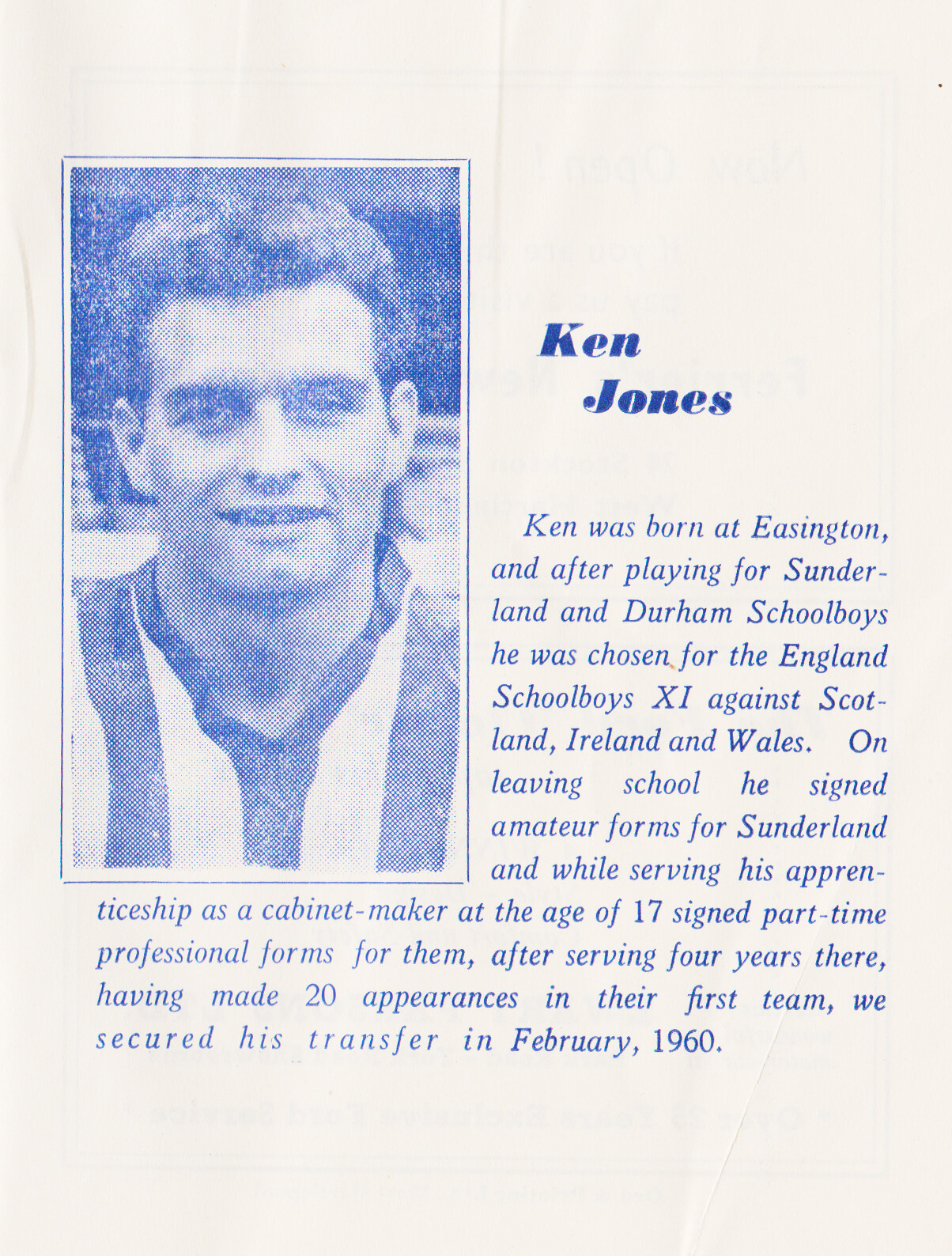The image depicts a scan of a slightly creased piece of light gray paper featuring biographical information on Ken Jones. On the left side is a blue and white pixelated photograph of Ken Jones, whose broad, smiling face with visible upper teeth and dark curly hair are prominent. He is donning a blue and white striped shirt. To the right of the photograph is a paragraph of text written in blue letters. The heading above this text reads "Ken Jones" and is divided into two lines. The biographical content details Ken Jones' journey from being born in Easington, playing for Sunderland and Durham schoolboys, to being chosen for the England schoolboys XI against Scotland, Ireland, and Wales. After leaving school, he signed amateur forms for Sunderland and at the age of 17 signed part-time professional forms while apprenticing as a cabinetmaker. The text concludes by noting that after making 20 appearances in Sunderland's first team over four years, his transfer was secured in February 1960.